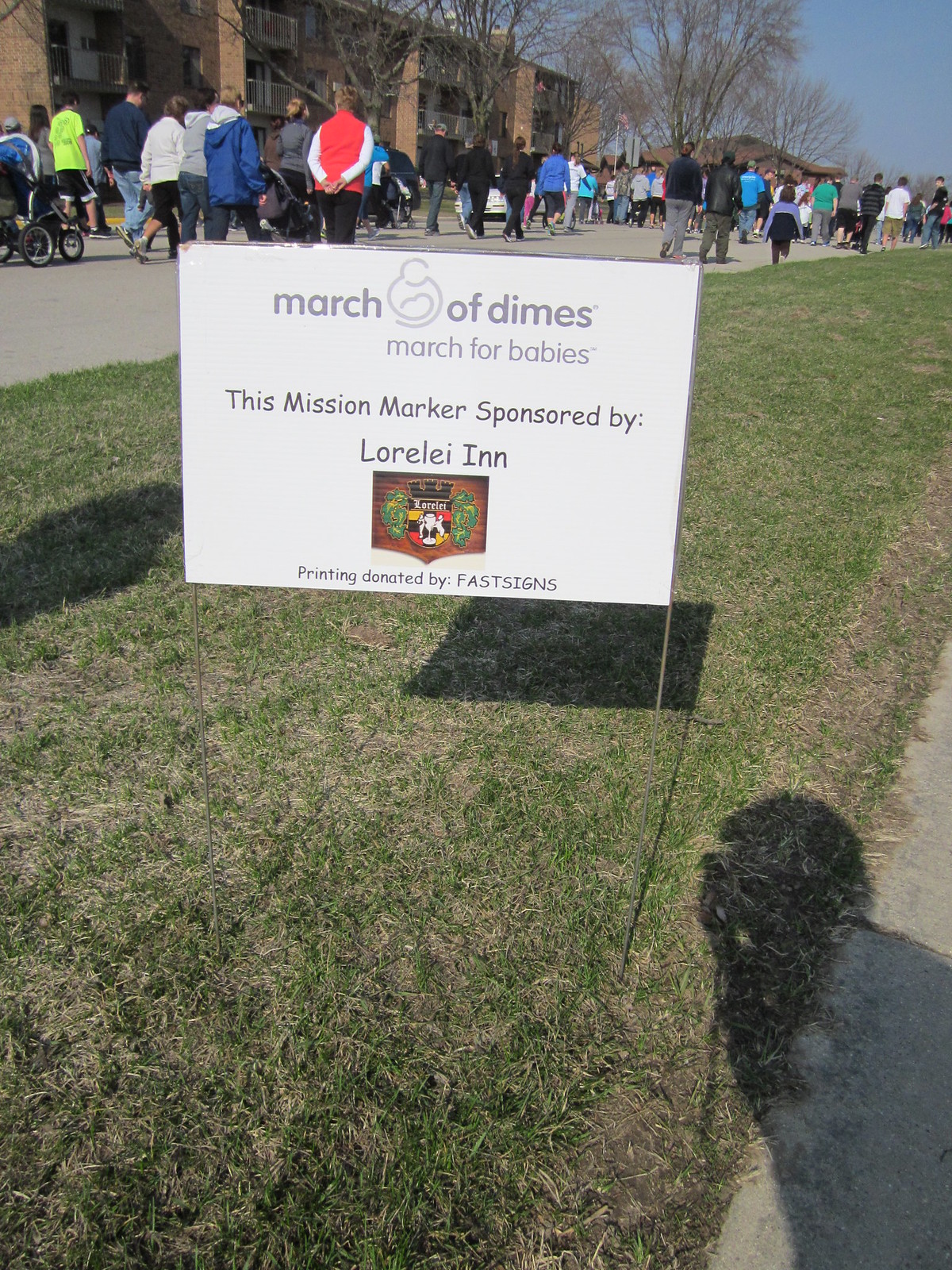This vertically aligned rectangular photo captures a vibrant scene from a March of Dimes, March for Babies event. In the foreground, a white sign stands on two narrow metal poles, situated on a grassy median that appears dry in patches. The sign reads "March of Dimes, March for Babies" in gray at the top, followed by "This mission marker sponsored by Laura Lee Inn" and "Printing donated by Fast Signs" at the bottom. In the center of the sign, there's an emblem resembling an Irish shield. 

Behind the sign, a crowd clad in colorful jackets and long pants—indicative of cold weather—walks away from the viewer, participating in the event. The background features a multi-level, brown and tan building to the left, and leafless trees with bare branches. A sliver of blue sky is visible in the upper right, adding to the crisp outdoor setting.